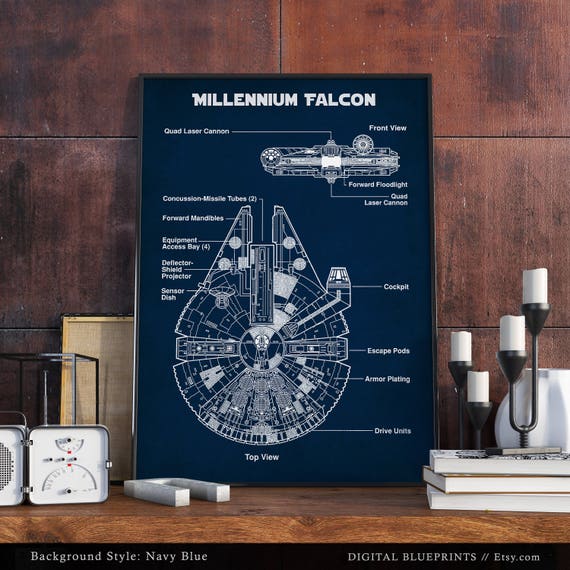This image appears to be a promotional or decorative photograph set in an office or living room. The central focus is a detailed, framed blueprint poster of the Millennium Falcon from Star Wars, displayed in a thin black frame. The diagram includes both a front and top view of the spaceship, accompanied by labels for each part. The blueprint itself is set against a navy blue background with the title "Millennium Falcon" prominently in white print. Along the bottom edge of the poster, a black strip reads "background style navy blue" and "digitalblueprints//etsy.com."

The framed poster is leaned up against a medium to reddish-brown wooden paneled wall and rests on a wooden shelf. To the right of the poster, there is a black candelabra with four thick white candles, positioned atop a stack of three books. To the left, there is a wire box and in front of it sits a small, old-school radio-like device with dials. At the base of the setup, a white magnet shaped like a traditional horseshoe magnet adds an additional element of interest to the scene. The overall arrangement gives a sense of curated decor that might be featured in a magazine or advertisement.